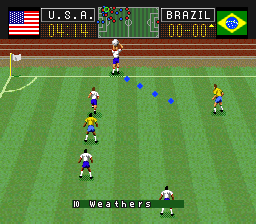This square digital image depicts a nostalgic scene from an old-fashioned video game, reminiscent of early Game Boy or similar retro gaming systems. The visuals are characteristic of simplistic, low-resolution graphics typical of that era. The image portrays a soccer match between the United States and Brazil on a large, green field.

To the left side of the field, there is a flag. In the background stands a scoreboard bearing the United States flag and displaying the text "USA." The main focus of the image is the detailed view of players represented as red and blue dots, indicating their respective teams against the green pitch. Brazil's team is identified by their flag on the right side of the scoreboard.

Positioned left of the center are three players who appear to be either running or standing, all facing towards the main player at the top-center of the image. This main player, distinguished from the rest, is holding a soccer ball. There are noticeable blue squares on the ground, creating a directional cue that points towards another player located on the right side, who is wearing a yellow shirt.

The players' uniforms consist of colors like yellow, blue, and white, clearly differentiating the teams: the United States players in blue and the Brazilian players in yellow. A small, dark green text bar situated towards the bottom of the image specifies "10 weathers," possibly indicating some in-game conditions or settings.